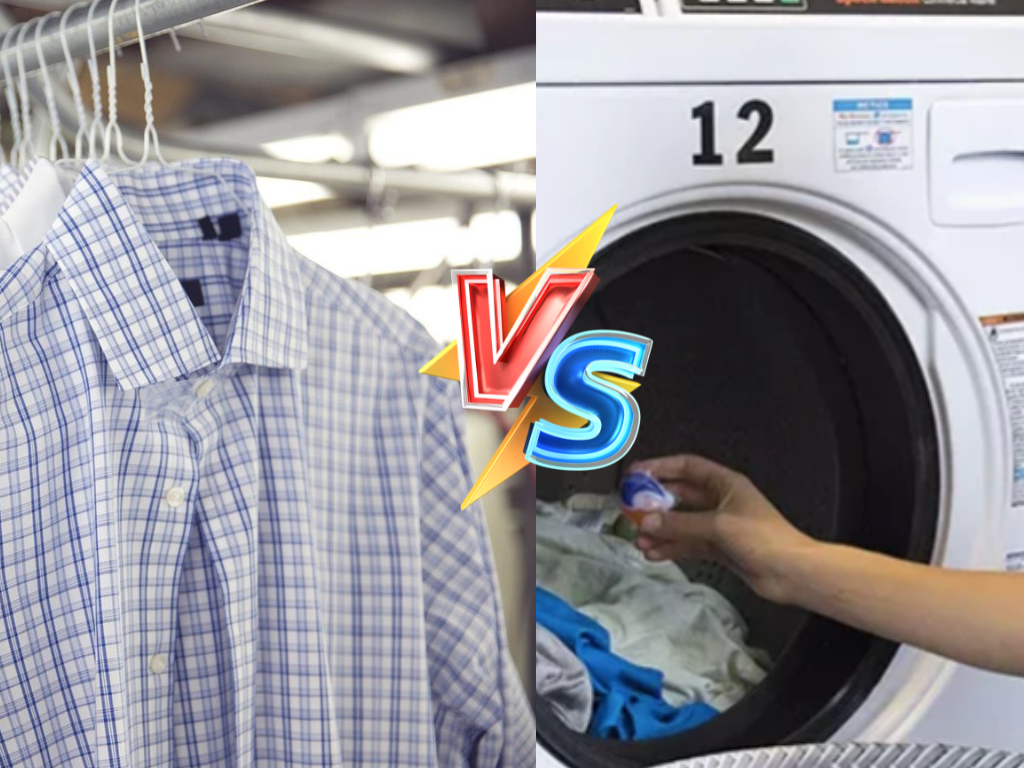The image is a split advertisement for laundry detergent pods, featuring a vivid central logo with a yellow lightning bolt and the letters "V" and "S" in neon-style, with the V in red and the S in blue. On the left side of the ad, there is a metal rack with white wire hangers holding several collared button-up shirts. The foremost shirt is a blue and white striped button-up, while another appears to have a plaid pattern. On the right side, an open laundromat washing machine marked with the number 12 reveals a mix of white, blue, and gray garments inside. A woman's hand is seen placing a detergent pod, blue on top and white at the bottom, into the washer's drum.